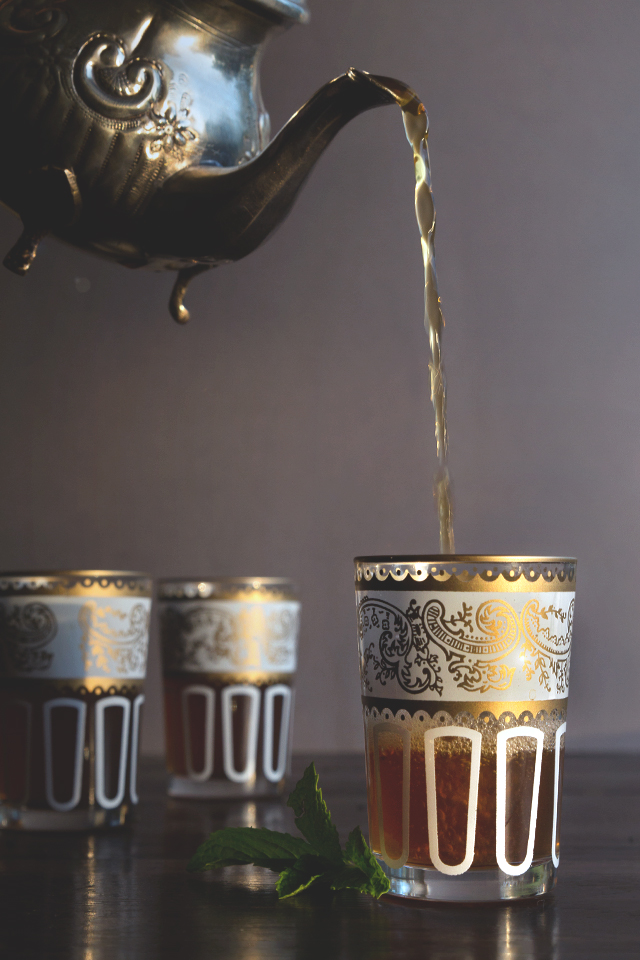In this softly glowing portrait-style image, a silver teapot with golden light highlights is pouring tea into an elaborate glass cup in the foreground on the right-hand side. The teapot dominates the upper right corner of the frame, featuring intricate designs. The glass cup being filled with tea is adorned with a mixture of white and gold decorative patterns, including paisley-type swirls and circles surrounding the rim. This cup is positioned on a dark gray surface, accompanied by a sprig of fresh mint. In the background to the left, two similar glass cups with corresponding decorative designs and simpler bases are slightly blurred, adding depth to the image against a light gray wall.